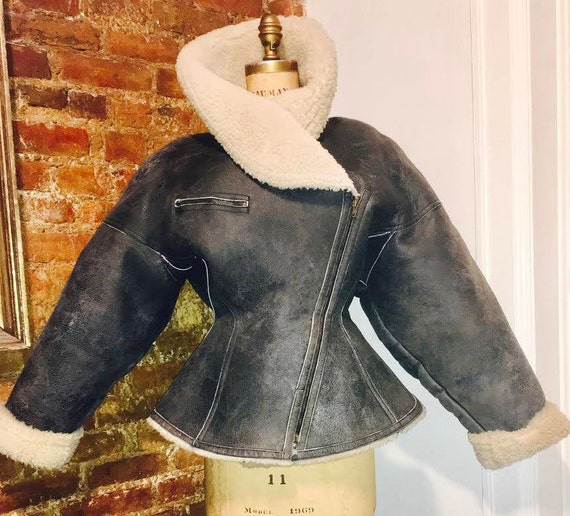The image depicts a vintage, distressed black leather jacket displayed on a tan dress form without a headpiece, situated against a background comprising a brick wall on the left and a very dark white, creamy surface that might be paneling or a door on the right. The jacket itself is waist-length and features a distinctive diagonal zipper running from the lower center to the upper right shoulder. It has a fur-like, cozy white fleece lining that extends to a prominent collar, which can either stand up or fold down to accentuate the fleece. The long sleeves of the jacket are turned up at the cuffs to reveal more of this white fleece, adding to its warm, snug appearance. A noticeable pocket with a zipper is positioned on the upper left side of the jacket as viewed in the image. The jacket and the dress form evoke a vintage aura with their wear and styling.